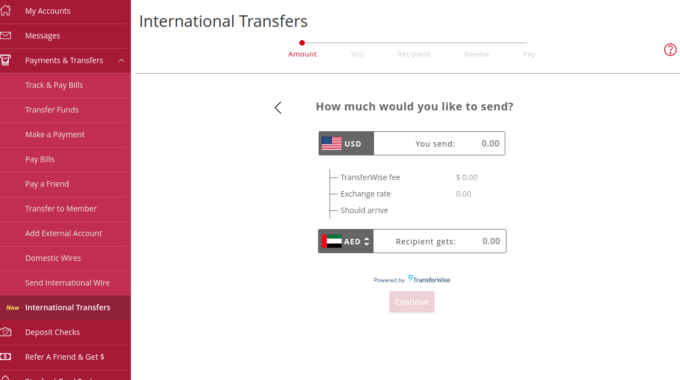The image is a detailed depiction of a financial app interface, divided into two primary sections: a navigation menu on the left and an international transfer screen on the right.

### Left Section: Navigation Menu
- **Background Color:** Pink gradient running vertically.
- **Top Section:** 
  - **Title:** "My Accounts"
  - **Icon:** Small house symbol on the left.
- **Navigation Options:** 
  - **Messages:** Envelope icon.
  - **Payments and Transfers:** "Track and pay bills, transfer funds, make a payment, pay bills, pay a friend, transfer to member, add external account, domestic wires, send international wire." 
- **Highlighted Section:** 
  - **Text:** "New" in yellow.
  - **Option:** International transfers.

- **Lower Section:** 
  - **Text:** "Deposit checks" with a camera icon.
  - **Referral Program:** "Refer a friend and get money" with a dollar bill sign icon.

### Right Section: International Transfer Screen
- **Background Color:** White.
- **Top Section:** 
  - **Title:** "International Transfers" in black.
  - **Divider:** Very faint gray line.
- **Middle Section:**
  - **Amount Section:** 
    - **Icon:** Red circle with "Amount" under it in red.
    - **Steps:** Labeled as "You", "Recipient", "Review", "Pay".
  - **Help Icon:** Red circle with a question mark.
  - **Prompt:** "How much would you like to send?" with a left-pointing arrow.

- **Sending Amount:**
  - **Currency Box:** 
    - **Flag:** American flag (gray).
    - **Label:** USD.
    - **Input:** "You send 0.00".
  - **Fee Information:**
    - **Label:** "Transfer-wise fee" followed by "$0.00".
    - **Exchange Rate:** "0.00".
  - **Arrival Time:** Labeled as "Should arrive."

- **Receiving Amount:**
  - **Flag:** With red, green, white, and black stripes (AED).
  - **Input:** "Recipient gets 0.00".
  - **Powered by:** "Powered by TransferWise" in very small font.
- **Action Button:** 
  - **Label:** "Continue" in white within a faint red box, indicating it's currently unselectable.

The overall layout presents a clean and functional user interface designed to facilitate international money transfers with clear steps and detailed options.